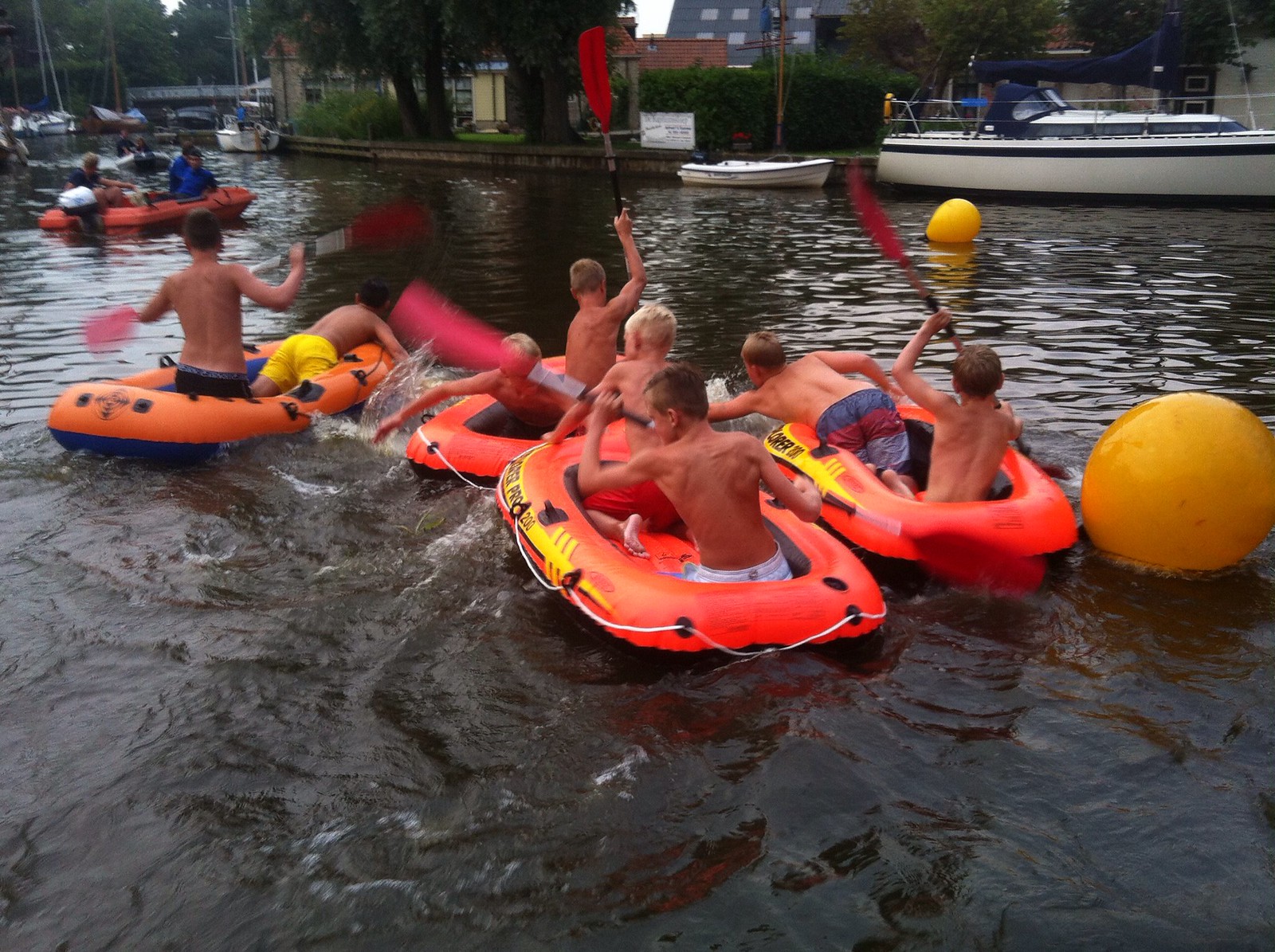The photograph captures a lively scene on a river where several young boys, identifiable by their short hair and bare torsos, are engaged in what appears to be a competitive activity in small, orange inflatable paddle boats. Each boat, resembling an inflatable life raft with blue or black bottoms, carries two boys. They are energetically paddling with double-ended red paddles attached to metal poles with black handles. The water is dark green and murky, with small splash waves visible from the boys’ movements. In the middle of the river, the boys seem to be either leaning forward, possibly jostling or reaching into the water, suggesting a playful yet competitive atmosphere. Surrounding the boats, there's a white string, potentially part of the competition setup. In the background, a larger motorized boat, also orange, has several people aboard observing the activities. Additional motorboats and a couple of yellow floating markers dot the scene, along with a shoreline covered in green bushes and big brown trees with lush green tops. The activity is bathed in daylight, contributing to the vibrant and energetic feel of the image.